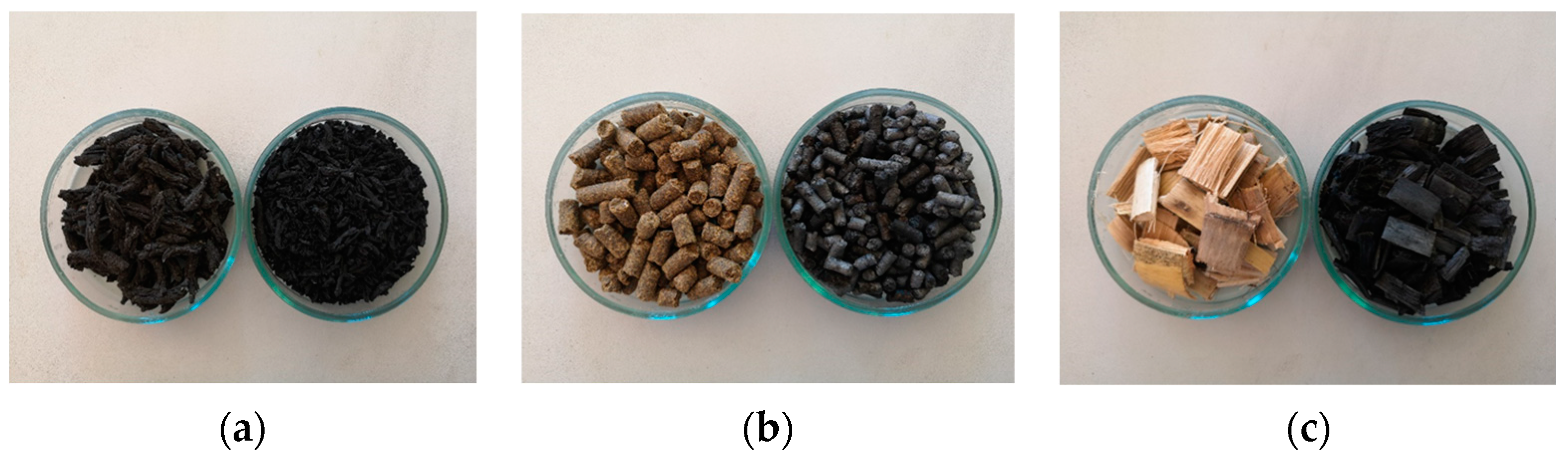The image is composed of three side-by-side sections labeled A, B, and C, each featuring two clear glass bowls filled with different substances. In section A, the left bowl contains a black, granular material resembling either black powder or a fine mulch, while the right bowl holds another type of black material that appears slightly more diced or granular. Section B features a brown, pellet-like substance in the left bowl and a black, similarly-sized pellet substance in the right bowl; these materials resemble types of animal feed. In section C, the left bowl contains light wood chips, and the right bowl contains what looks like chunks of charcoal. Each section showcases the contrast between two distinct substances placed in transparent bowls for clear visibility.